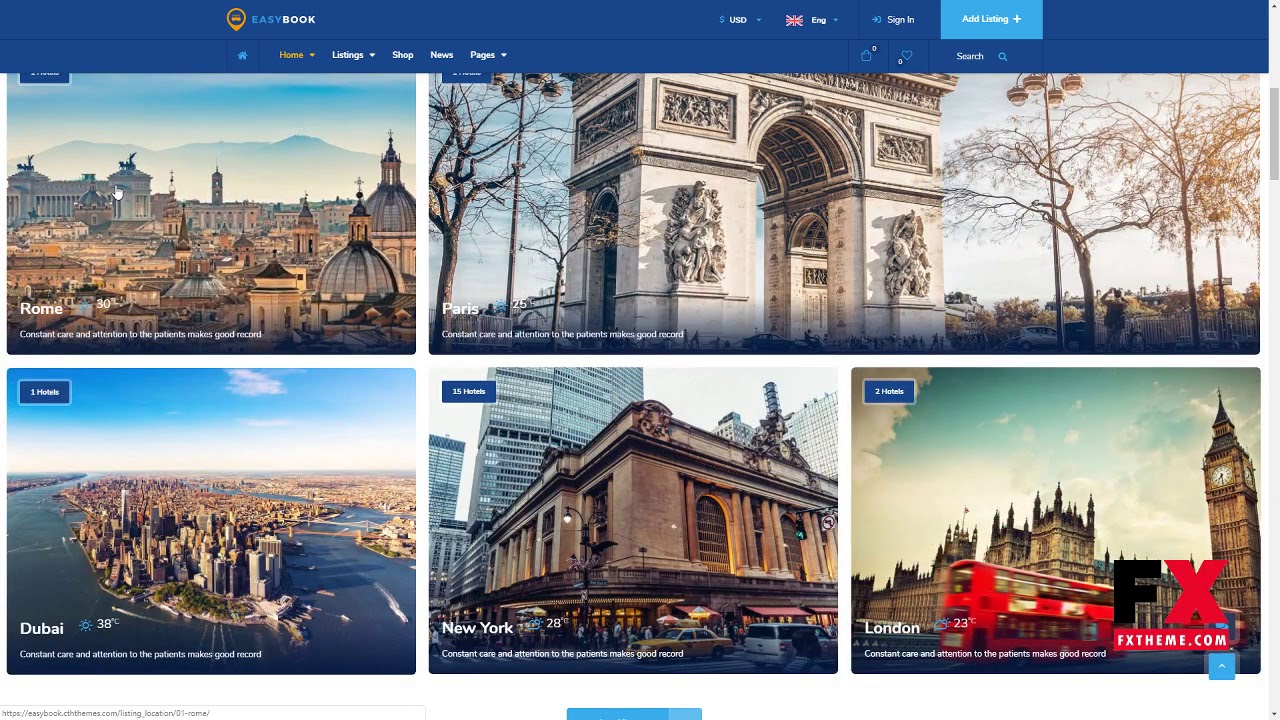This screenshot captures a user interface of a travel booking website featuring a dominant dark blue banner at the top. The rectangular image, which is longer horizontally, includes various elements that contribute to its functional and aesthetic design.

In the upper left corner, the brand name "Easy Book" is prominent, accompanied by a logo to its left featuring an orange design with a small orange car. Towards the upper right corner, the currency symbol "USD $" is displayed, followed by an icon of the UK flag and a "Sign In" button.

Below this banner, a horizontal menu extends from left to right, featuring icons and text for navigation. Starting from the left, there is a home icon beside the word "Home" in yellow text with a pull-down arrow. Next to it are tabs labeled "Listings" with a pull-down arrow, "Shop," "News," and "Pages." Situated on the far right of this menu is a search bar, identifiable by a magnifying glass icon.

The main content area showcases five colorful photographs representing different cities. The upper left image presents a picturesque view of Rome, with "Rome" written in white text. Adjacent to it on the right, a daytime view of Paris is labeled with the city name in white block letters. 

In the lower left corner, an aerial perspective of Dubai displays the temperature reading "38 degrees Celsius" along with smaller text beneath that reads, "Constant care and attention to the patients makes good record." Following Dubai, the next city featured is New York, and finally, London is displayed to the right, completing the collection of city images.